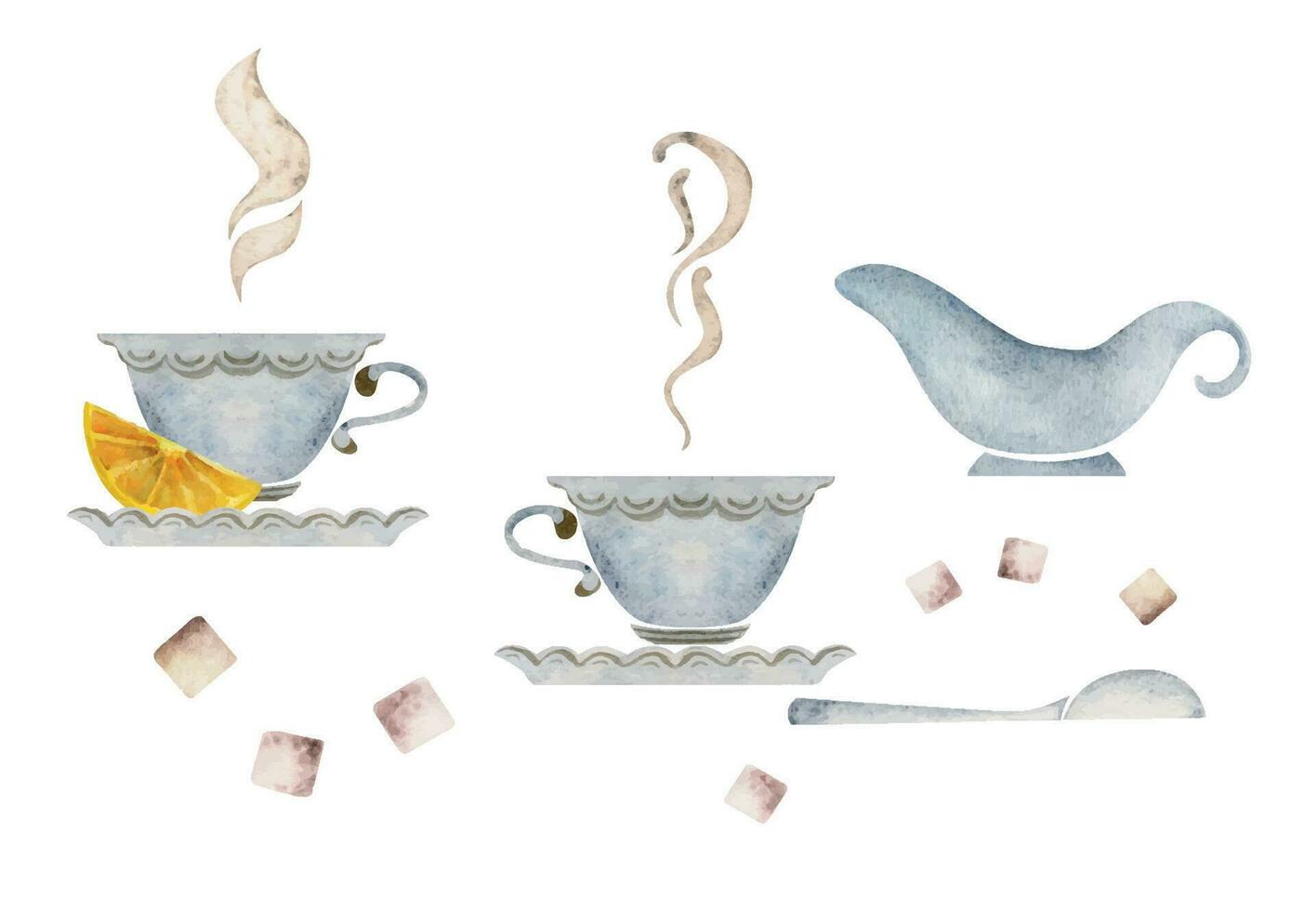This is a detailed, cartoonish drawing featuring two stony gray, finely crafted teacups with curly handles, both emitting steam, sitting on gray saucers. One teacup, with its handle pointing right, sits adjacent to a slice of orange on its saucer. The other teacup, with its handle facing left, mirrors the style and color. Scattered around the scene are seven sugar cubes rendered in shades of white and brownish-gray. Towards the bottom right, there is a gray, bathtub-shaped serving ladle, accompanied by a matching serving spoon, which lies face down with its concave part facing the ground.